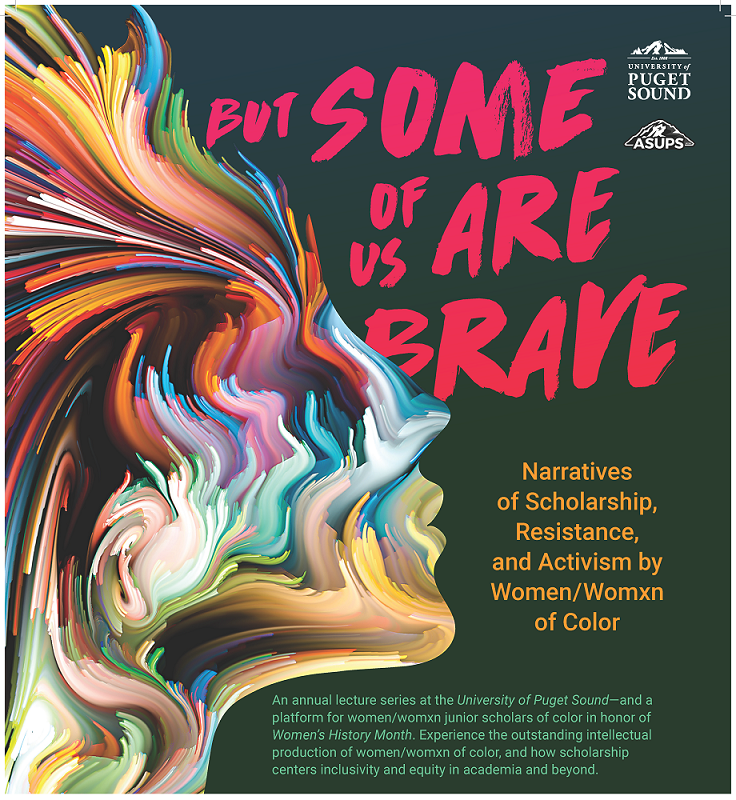This vibrant poster, set against a green background, advertises an annual lecture series at the University of Puget Sound titled, "But Some of Us Are Brave," with the phrase appearing in prominent pink text. Spearheaded by the University and ASUPS, the series celebrates Women's History Month by showcasing narratives of scholarship, resistance, and activism by WOMXN (an inclusive term for women) of color. The poster also mentions that it serves as a platform for junior scholars of color, highlighting the theme of inclusivity and equity in academia. The left side of the poster features an eye-catching, multicolored side-view portrait of a woman, with hues of blue near the nose, reds around the eyes, and greens, pinks, and yellows in the hair, creating a striking rainbow effect. At the top right, the university's name, "University of Puget Sound," is displayed.